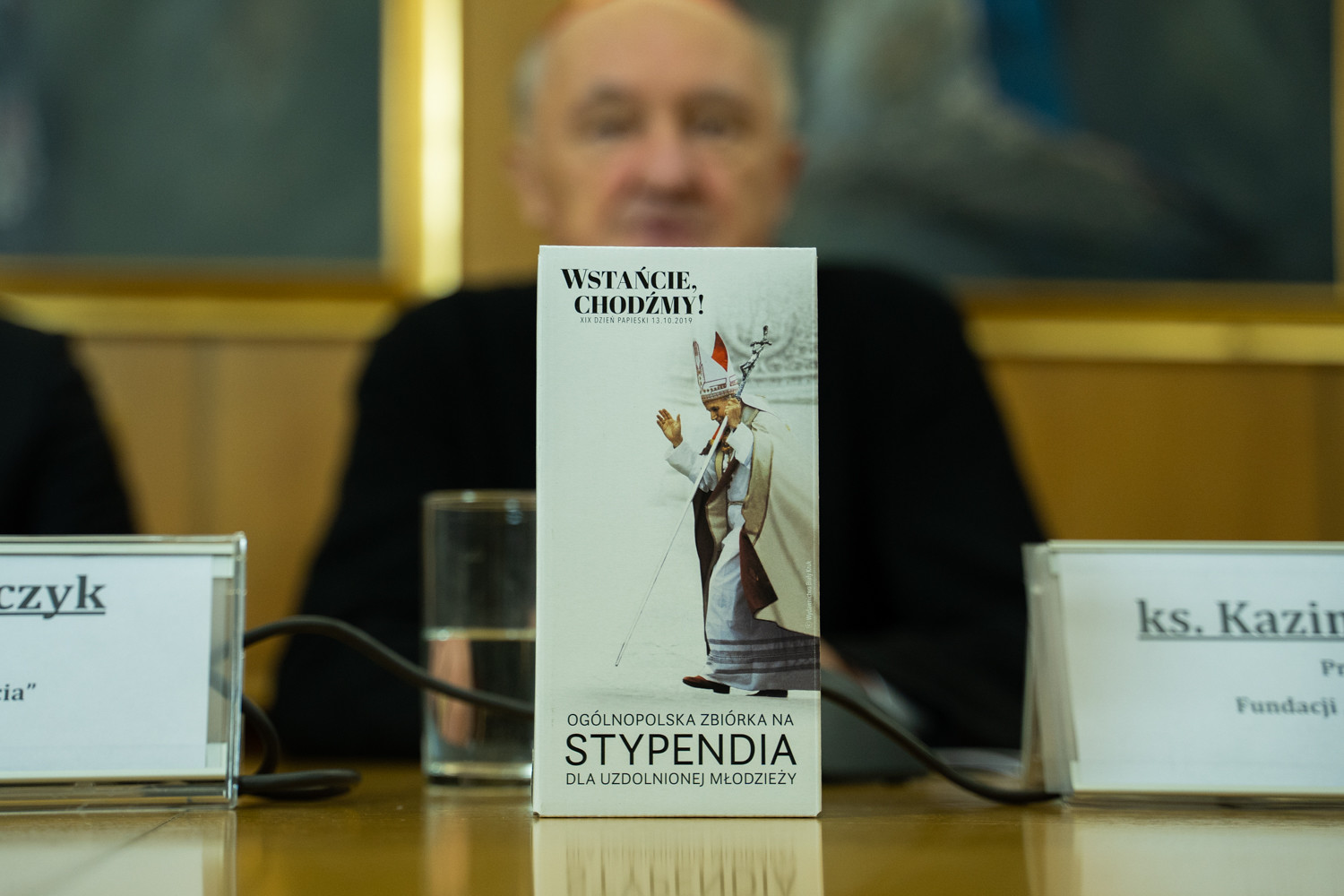The image depicts an older man with white hair on the sides of his head, wearing a dark sport coat or sweater, seated at a table with a microphone and a glass of water in front of him. Dominating the foreground is a paper placard or booklet standing on the table, featuring an image of the Pope dressed in a long white robe with a beige cape, a tall white hat with red detailing, and holding a walking stick topped with a crucifix. The text on the placard is not in English: it reads "W-S-T-A-N-C-I-E C-H-O-D-Z-M-Y" at the top and "O-G-O-L-N-O-P-O-L-S-K-A Z-B-I-O-R-K-A N-A S-T-Y-P-E-N-D-I-A D-L-A U-Z-D-O-L-N-I-O-N-E-J M-K-O-D-Z-I-E-Z-Y" at the bottom. The event seems to be focused on the release of some media, possibly books or video cassettes. Everything behind the placard and the man, including additional signs with partial text "C-Z-Y-K" and "K-S. K-A-Z-I-R," is out of focus, emphasizing the placard and the man as the main subjects of the image.